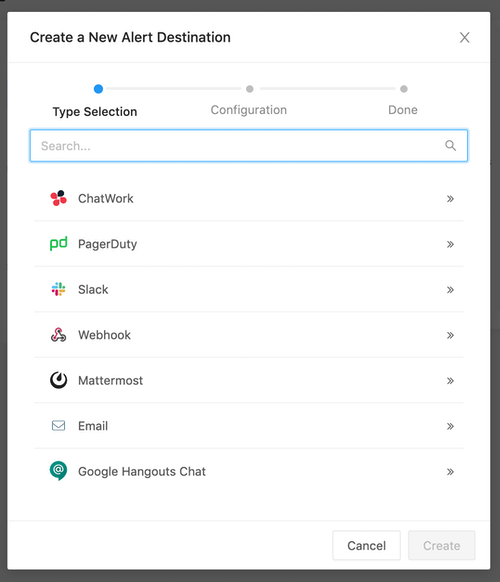Screenshot of a Website: Interface for Creating a New Alert Destination

This screenshot displays a clean and minimalistic user interface, likely from an organizer program or app, optimized for both mobile and desktop devices. The layout is designed to be user-friendly with a straightforward structure and minimal clutter, making it easy to navigate and read.

The primary function of the page is to facilitate the creation of a new alert destination, organized into three progressive steps:

1. **Type Selection** (currently active phase)
2. Configuration
3. Completion

At the top, there is a search function bar to help users quickly find specific options. In the "Type Selection" stage, a variety of alert destination types are listed, each accompanied by its respective icon on the left. The available options include:

- Chat Work
- PagerDuty
- Slack
- Webhook
- Mattermost
- Email
- Google Hangouts Chat

Each type provides a visual and textual identifier, making it simple for the user to choose the appropriate alert destination.

Overall, the interface exudes a modern and streamlined aesthetic, prioritizing ease of use and clarity for an efficient user experience.